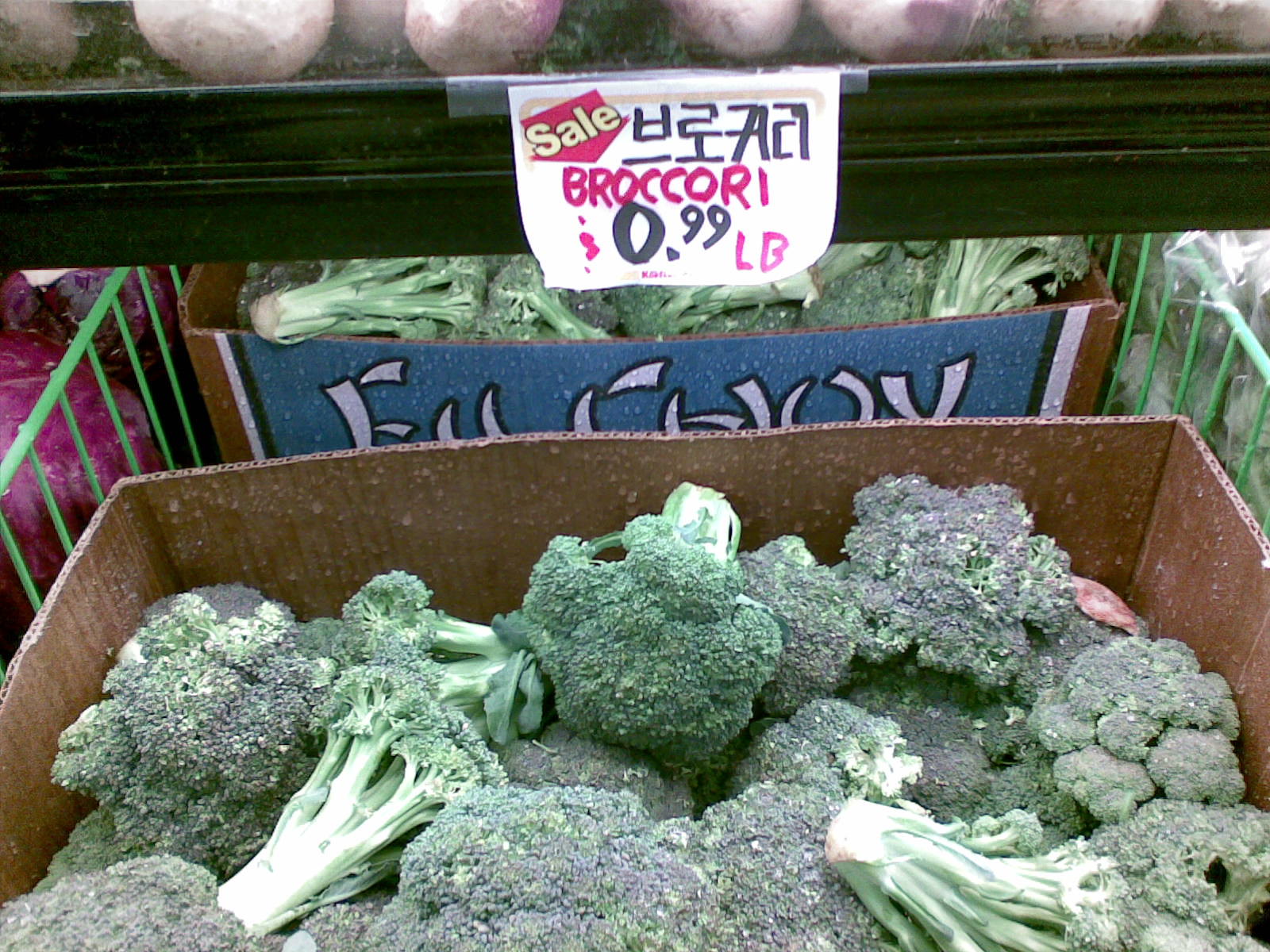This photograph depicts a market scene focused on a cardboard box filled with broccoli crowns, prominently marked with a white tag indicating a sale price of 99 cents per pound. The sign features both an Asian language and the English word "broccoli," hand-written in marker. Behind the main box, there is another box similarly filled with broccoli, nestled beneath a shelf. Above the boxes, the shelf is partially visible and appears to hold purple and white turnips. To the left of the broccoli box, partially visible, are what seem to be red cabbages, while to the right, there is an indistinct green vegetable encased in plastic packaging. The boxes of broccoli and adjacent vegetables are separated by green metal wire dividers that organize the shelf space.